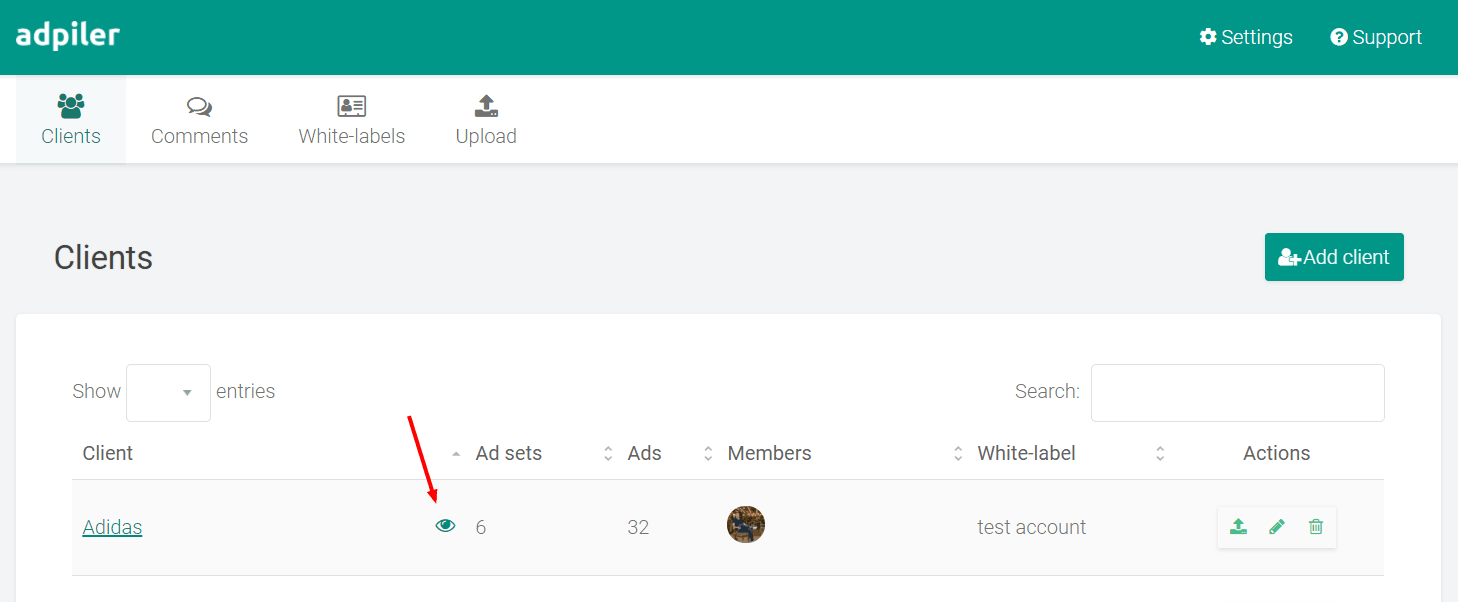Screenshot of a computer monitor displaying an application interface:

At the top of the rectangular image is a dark green horizontal bar with text elements and icons. On the upper left corner, in white lettering, it says "ADD PILAR." On the right corner of the green banner, there is a white settings gear icon next to the word "Settings" in white. Additionally, there is a white circle containing a question mark labeled "Support."

Below the green banner, the background alternates between white and gray. Directly beneath the banner, in white text, it says "Clients" with an icon of a person to its right. This is followed by "Comments" with a speech bubble icon above it, "White Labels" with a Rolodex-type card icon above it, and "Upload," represented by a black bar with a gray up arrow.

In the gray section below, it says "Clients" again, this time in dark gray text. On the far right of this section, there is a green button with white text that says "Add Client."

Beneath this, there is a section with a dropdown labeled "Show" for selecting the number of entries to display, followed by the word "Entries" on the right. The main content area lists multiple columns: the first column labeled "Client Adidas," which appears as a hyperlink. The second column is labeled "Ad Sets" and displays an eyeball icon with the number 6 and a red arrow pointing down toward the eyeball. The third column is labeled "Ads" and shows the number 32. The fourth column is labeled "Members" and contains a dark-colored, indistinct icon. To the right of this, there is a label that reads "White Label Test Account."

On the far right, there is a section labeled "Actions," containing three icons: a green person, a pencil, and a trash can.